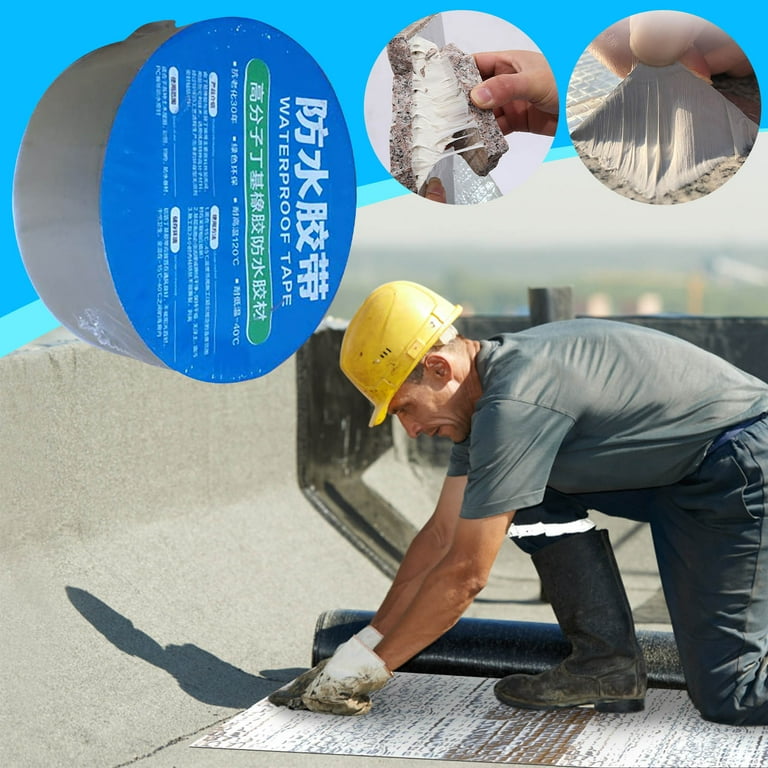The image is a square-shaped advertisement for waterproof tape. At the top of the advertisement, there is a bright blue band featuring a gray roll of tape with a blue label containing white lettering, which indicates its waterproof nature. The roll also includes Chinese lettering, which suggests the product's origin or additional instructions. To the right of the tape, within the blue band, there are two circular inset photographs depicting the application method for the tape, showing a person pulling the tape off, indicating its strong adhesiveness.

Below the blue band, a construction worker is prominently featured. He is wearing a yellow helmet, a gray shirt, dark pants, boots, and white gloves. The worker is crouching down, focused on applying the waterproof tape to something on the ground. This primary photograph vividly demonstrates the practical use of the tape, enhancing the advertisement’s message.